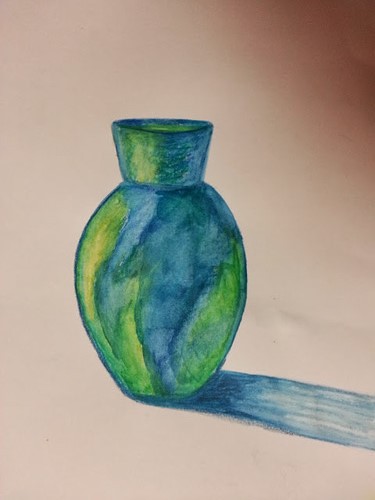This still-life drawing, set on very light brown cream-colored paper, features a prominently detailed vase. The vase, positioned at the center of the image, occupies about half of the composition. It displays a subtle, oblong shape with a sphere-like body and a smaller, somewhat spherical opening at the top, which flares out in a cup fashion. The vase is a blend of aquamarine blue and various shades of green, including light and yellow greens, with streaks and striations that mimic the appearance of continents on a globe. Adding to the intricate design, the vase is outlined in a darker blue pencil.

The vase casts a thoughtfully rendered shadow off to the bottom right side of the paper, indicating a light source from the left. This shadow shares the vase's blue tones, starting darker near the vase’s base and gradually lightening towards the edge of the paper. Additionally, the background transitions from off-white to a darker brown in the upper right corner, possibly from a cast shadow, further enhancing the depth and realism of the composition.